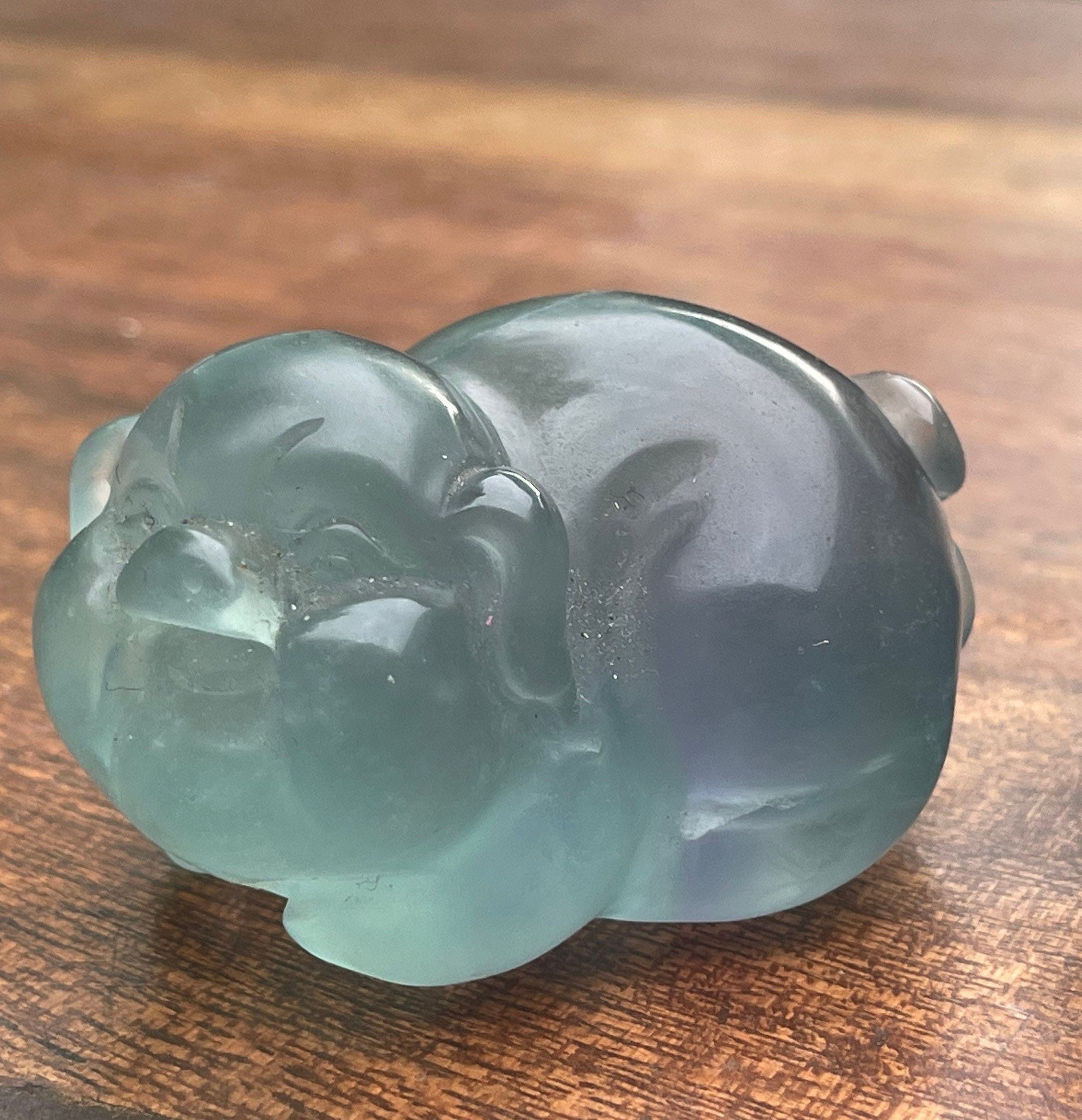The image showcases a detailed, close-up view of a glass sculpture resembling a small pig. The pig is crafted from opaque, teal-colored glass, appearing almost bluish-gray. The material gives it a reflective quality, contributing to varying shades of blue across its body. The pig’s round body features a distinct curled tail and a large, smiling face with big cheeks and a flat snout angled towards the left. The sculpture is intricately designed, with one front leg visible. It sits on a brown, wooden tabletop with a textured, notched surface that displays scratchy marks and lighter material in certain areas. The wood is slightly blurred in the upper background, ensuring the focus remains on the whimsical glass pig that seems to embody a playful and cheerful demeanor, reminiscent of an Asian cartoon style. The image is centered solely on this charming figure, with no additional text or people present.